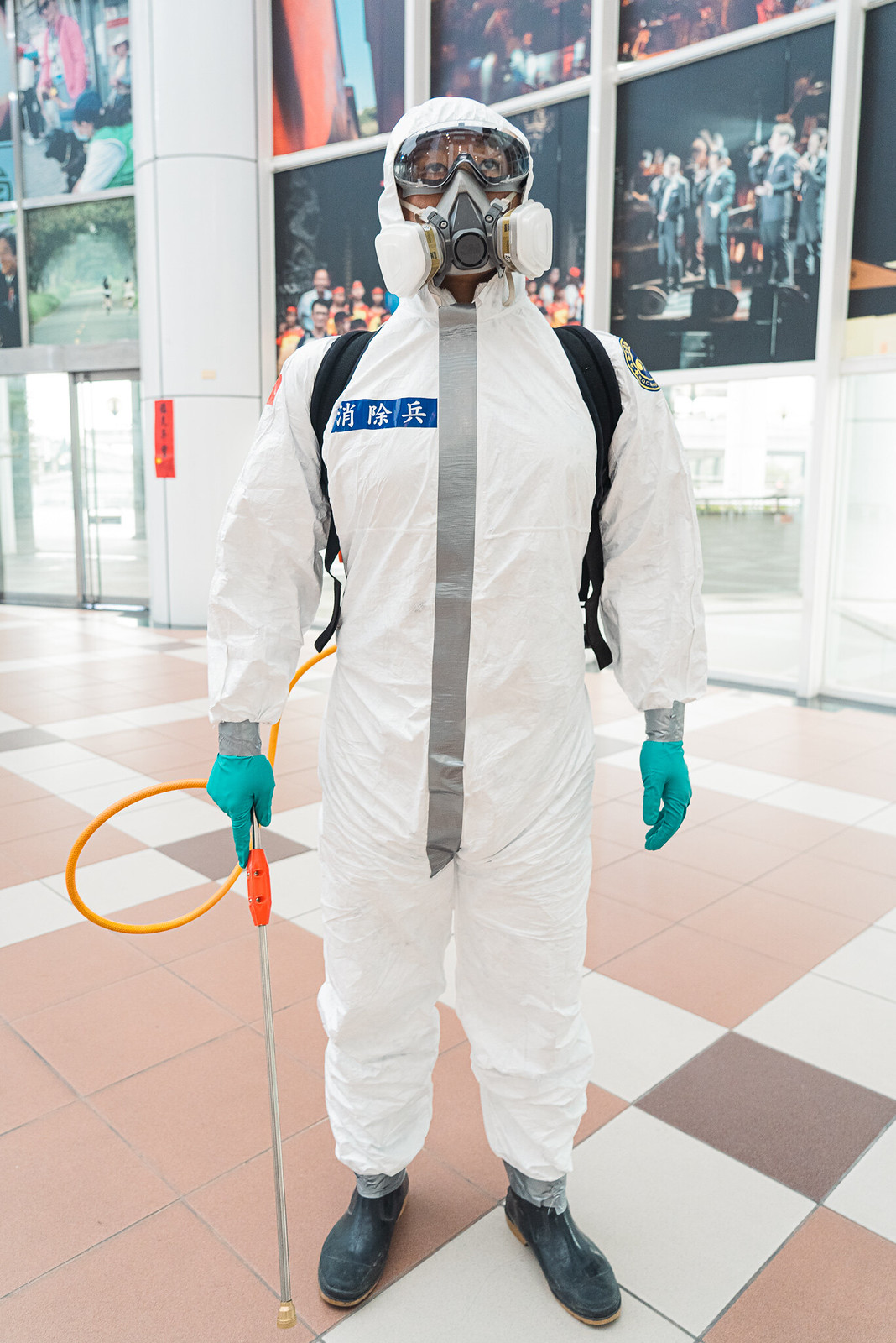This is a vertically aligned rectangular image featuring a man in a one-piece white hazmat suit. The suit includes a white hood that covers his head, a gas mask on his face, and goggles protecting his eyes. His ankles are meticulously taped around the suit to prevent any contamination. There is a blue strip of fabric with white, non-English symbols on the right chest area of the suit. He is also wearing blue nitrile gloves on his hands and black boots. 

In his left hand, he holds a yellow cord that is attached to an orange handle, which resembles the bottom of a cane and is part of a spraying apparatus. The hose from this apparatus extends from a backpack he is wearing, likely containing an oxygen supply or tank for spraying disinfectant. There is masking tape covering the zipper of his suit, from his neck down to his crotch.

The man is standing on a tiled floor with sections of brown, white, and dark brown square tiles. The environment appears to be a large room or building, possibly an auditorium or a performance art space, as suggested by the background, which features several large posters that look like they're of musicians. Glass doors can be seen to the lower left side, suggesting an entranceway or lobby area.